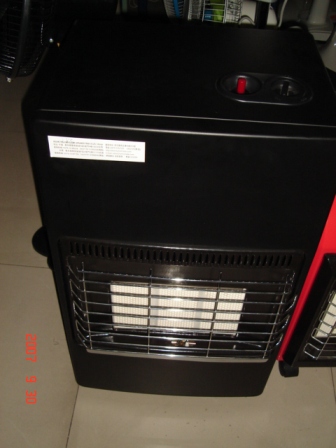This image depicts an ambiguous black vertical rectangular device standing on a gray-tiled floor, surrounded by shelving and other indistinct products, suggesting a store setting. The device is approximately four feet high, with a distinctive design that includes a red switch on the upper right corner of its top and appears to have additional switches or buttons. A white label with black text is visible on the upper front section, but it's too small to read clearly. Below the label, the device has a ridge that protrudes slightly, followed by a silver grill composed of multiple vertical and horizontal metal rods. This grill covers a white section, which could either be a component related to heating or part of a window into another function like shredding. The exact purpose of the device remains ambiguous; it could be a portable heater or possibly a paper shredder.